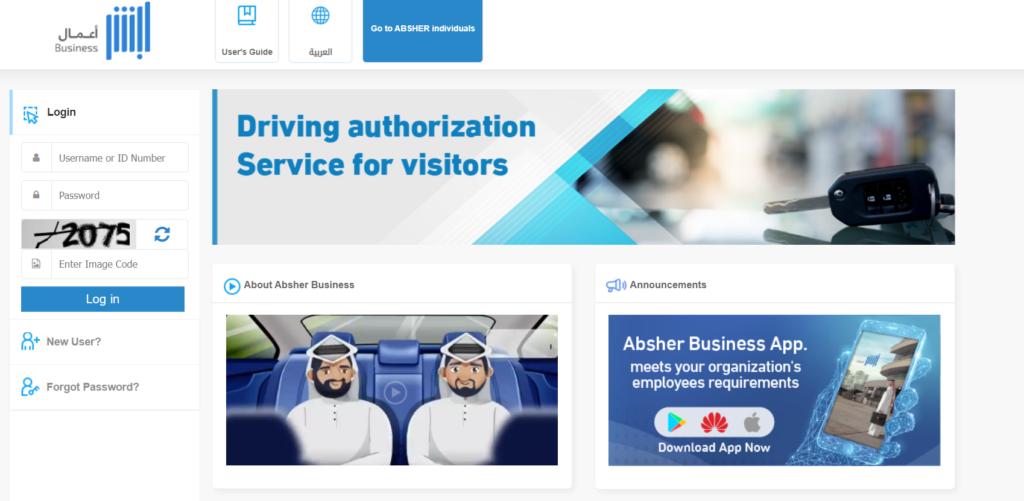In the upper left corner of the image, there is a black text reading "Business" accompanied by some Sanskrit text above it. Below this, there are six horizontal lines, three of which have dots above them, and one has a dot below, all rendered in blue. Moving to the right, it reads "User's Guide" followed by more Sanskrit text and an icon symbolizing a globe. Further right, the letters "A, B, S, H, E, R" spell out "Abshir Individuals."

In the left section below, there's a vertical navigation menu. The top item says "Login," followed by fields labeled "Username or ID" and "Password." Beneath these fields, there's the number "2775" and a refresh button next to it, accompanied by a field labeled "Enter Image Code." Below these inputs are links for "New User" and "Forgot Password."

In the middle section of the image, the text "Driving Authorization Services for Visitors" is displayed in blue on a grey background. Below this text is a photograph featuring a car key, likely with an integrated key alarm.

Towards the bottom right, two horizontally elongated rectangular images are positioned side by side. The images show two Middle Eastern men dressed in white, seated in the backseat of a car with blue upholstery.